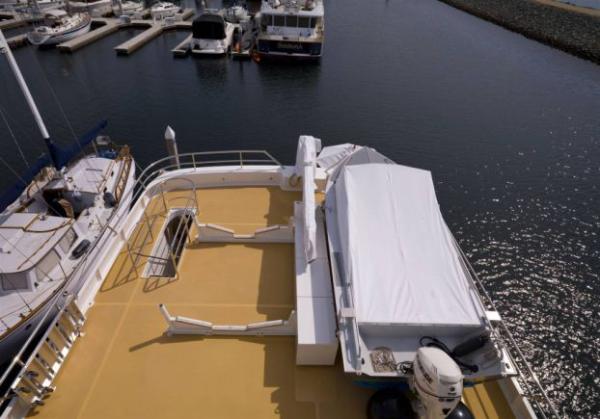The vivid color photograph captures a sunny day at a marina, characterized by a top-down view of a large, partially visible boat docked within the marina's bounds, possibly engaged in some renovation or construction work. This large boat, only visible from its rear half, is positioned prominently in the foreground on a flat, tan-colored deck that is devoid of any furniture or seating. An intriguing feature is the staircase situated in the top left corner of the deck, encased by a rounded railing, that leads below deck. The deck also contains a frame designed to hold two boats, although currently it cradles just one—a small white motorboat or dinghy equipped with an engine. On the right, the sun reflects off the serene blue water, bordered by a stone square wall visible in the top right corner. Surrounding the central boat are multiple other small and medium-sized boats docked in the marina, with several empty slips indicating available space. The composition includes a color palette of brownish tan, white, blue, gray, and black, with the photograph capturing the busy yet tranquil ambiance of the marina atmosphere.